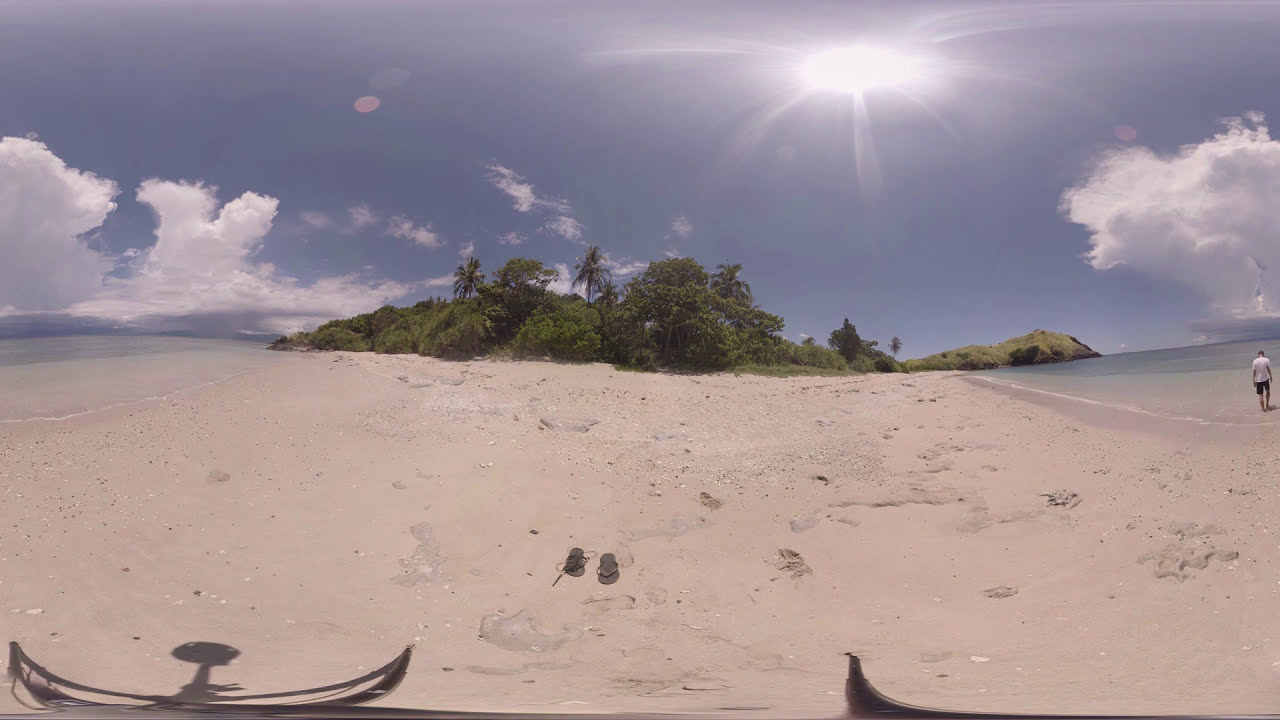This panoramic image captures a serene beach scene with intricate details throughout. In the foreground, a pair of black flip-flops rests on the sandy beach, which has a unique pinkish-gray hue. Directly ahead, a dense cluster of palm trees and green foliage forms a lush barrier that frames the scene. To the right of this greenery, there's a large rock formation, also tinged with green. The beach extends to both sides, bordered by calm, clear water that gets progressively bluer as it stretches out to sea.

Towards the far right of the image, a man wearing a white shirt and dark shorts walks towards the gentle waves breaking on the shore. The sky above is a gray-blue light, accentuated with clouds converging towards the center, creating a dramatic backdrop. The sun, seen near the top right of the image, emits visible beams, slightly distorted due to the panoramic capture. Adding to the intricate details, the left bottom corner of the image reveals a shadow, likely cast by the camera that captured this panoramic view.